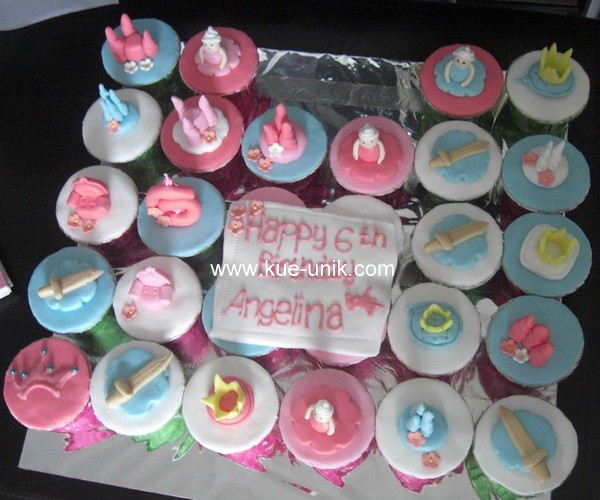The image displays a color photograph of 28 cupcakes arranged on a surface partially covered with aluminum foil and white paper, all set against a black background. The cupcakes are organized in a grid format with one row of four and six rows of four, forming a square-like structure akin to a birthday cake. Each cupcake features pastel-colored frosting in pink, blue, and white. The toppings on the cupcakes are intricately made of fondant and include various shapes such as crowns, swords, tiny castles, pink armchairs, and princess figures. In the center of the arrangement, there is a white fondant square bearing the message "Happy 6th Birthday, Angelina" written in pink icing. Superimposed across the middle of the image, a white watermark reads "www.kue-unik.com." The cupcakes appear to be homemade, with some frosting and other decorations spilled onto the surface below.